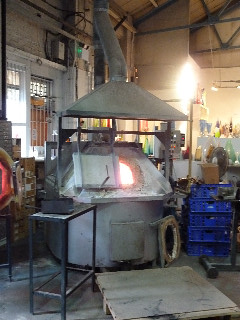This very small, rectangular photograph, measuring approximately 2 inches by 3 inches, depicts an indoor workshop scene. Dominating the center of the image is a large cylindrical metal furnace or kiln with its door half-open, revealing a hot, white fire burning inside. Above the kiln, a ventilation hood and pipe system snakes upward, presumably to release smoke outdoors. The workshop, which has high ceilings typical of an older warehouse, features barred windows on the left, allowing bright daylight to flow in. Fluorescent lights hang from above, adding to the illumination. There is a gray, concrete floor with a metal table and a platform to stand on in front of the kiln. On the right side, there are five blue crates stacked near shelves filled with various objects, including what appears to be blown glass, suggesting that this kiln is used for heating glass. The walls are cream-colored, and an industrial fan is mounted to the left side wall. The scene is devoid of people and any date indications, capturing a quiet moment in what seems to be a glass-blowing workshop.